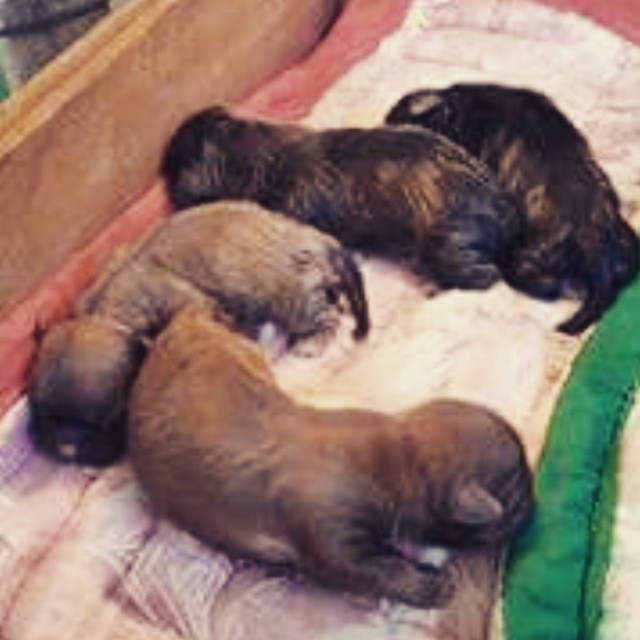In this overhead photograph, four newborn puppies are nestled together in a semicircular arrangement, creating an endearing, cozy scene. Closest to the camera is a medium brown puppy laying sideways, its head facing right. Beside this puppy is a lighter brown companion, its head resting near the other’s rear, creating an intimate cuddle. Behind them, two darker brown puppies with light brown patches snuggle closely, one of them blending into the group with its head tucked behind its sibling. These tiny puppies, possibly Shih Tzus with their wet fur, triangular ears, and long tails, rest securely within a whelping box. They lie on an inviting white blanket with green and red trim, contributing to a homely atmosphere. The image hints at a wooden box as part of their enclosure, reinforcing their vulnerable and newborn state. The overall scene, though slightly grainy, captures the tender early moments of these tiny lives.